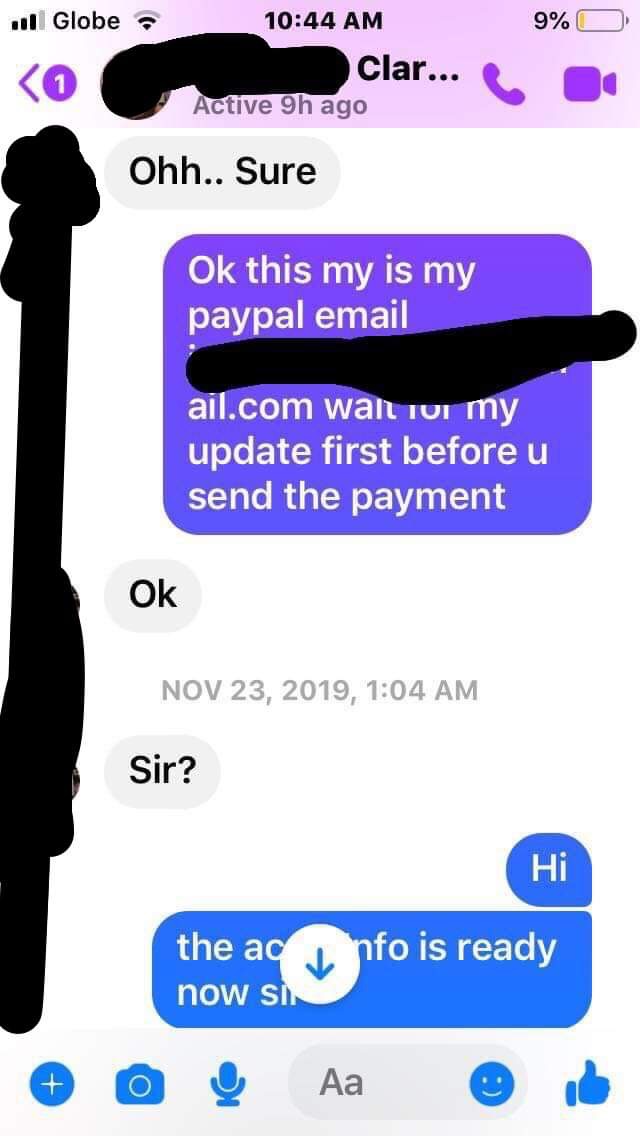This image captures a detailed screenshot of a text message exchange within a messaging app, likely Facebook Messenger. At the top of the screen, the status bar shows the user is on the Globe network with 3 out of 4 signal bars visible, accompanied by a 9% battery indicator. The time displayed is 11:44 AM. The sender's full name is partially obscured, showing only the letters "CLAR" followed by an ellipsis, and a greyed-out section indicates the name has been blacked out. Below this, it states "Active nine hours ago." 

On the right side of the screen, icons for a phone and a webcam can be seen. The main body of the screen shows a conversation where the initial message from one party states: "Oh sure." The subsequent response from the other participant is in white text on a purple background, reading: "Okay, this is my PayPal email," followed by blacked-out text, and continues with, "wait for my update first before you send the payment." The initial party simply replies, "Okay."

Following a timestamp of November 23, 2019, at 1:04 AM, the next part of the conversation starts with the initial party stating, "Sir," to which the respondent answers, "Hi." The final visible message says, "The account info is ready now, sir," though part of this message is blocked.

At the bottom, various icons for adding someone, viewing photographs, using a microphone, inserting a smiley, and sending a thumbs-up are displayed, all colored blue. There is an evident blackout stripe alongside the left edge, likely covering user or profile images.